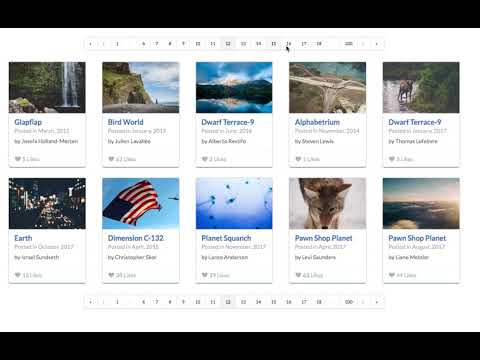A small webpage serves as a repository for a variety of stunning images, arranged in two rows of five. Each image is accompanied by a unique and somewhat cryptic description that doesn't quite match the visual content. The images predominantly showcase outdoor scenes and are professionally photographed. Among the striking visuals, there's a majestic waterfall, a mysterious cave near the coast, and a place labeled "Dwarf Terrace," whose exact nature is unclear. Another image, titled "Alpha Betrium," depicts a mining operation. An additional "Dwarf Terrace" is present, displaying an outdoor shot near a river. A nighttime street scene bustling with cars is labeled "Earth." Another captivating image shows the American flag waving against a sky backdrop declared as "Dimension." A photograph of a coyote bears the enigmatic title "Pawn Shop Planet." The unusual names and the high-quality photography give the impression that these images and captions might be placeholders used for testing the site.